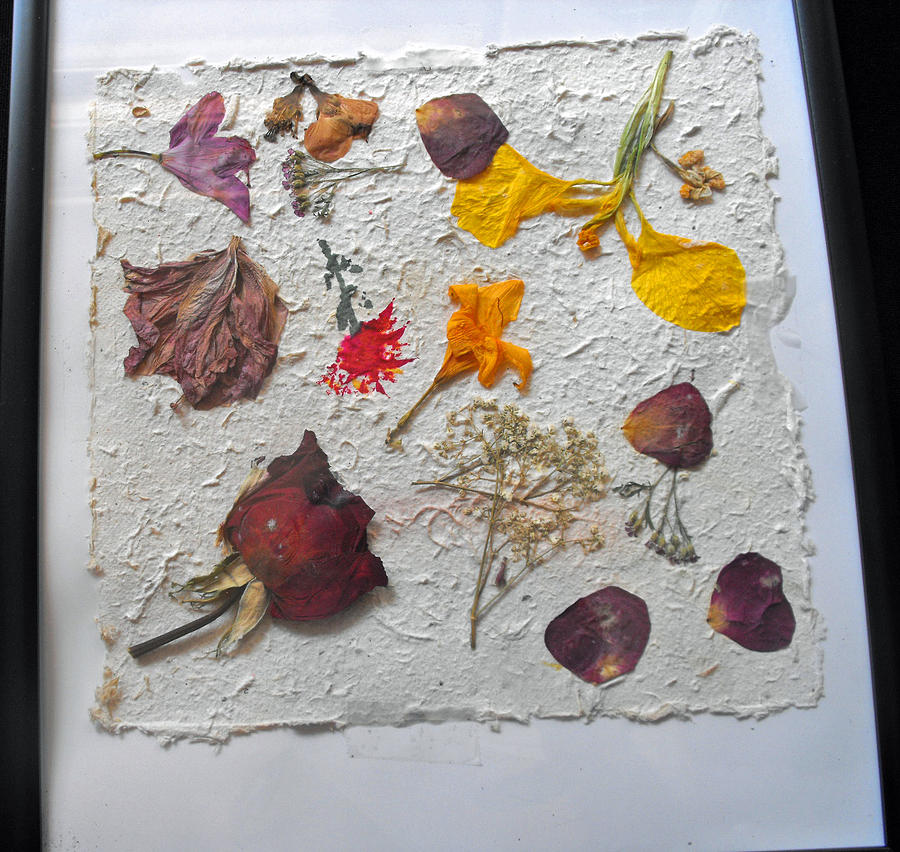This image showcases a beautifully framed arrangement of pressed flowers. The frame is sleek and black, complemented by a clean, white matting that provides a crisp backdrop for the delicate display. The flowers are pressed against a textured paper, which forms the central canvas for the arrangement. 

Within the frame, a vibrant red rose stands out, accompanied by a couple of its scattered petals. There is also a vivid yellow flower, an orangish-yellow blossom, and a striking purple flower, each meticulously pressed to retain their natural beauty. Adding an artistic touch, a red flower with a green stem, seemingly painted on, is included in the array.

The paper holding these flowers is neatly secured to the matting within the frame, though a few pieces of scotch tape can be seen, hinting at the careful handiwork involved in creating this botanical artwork.